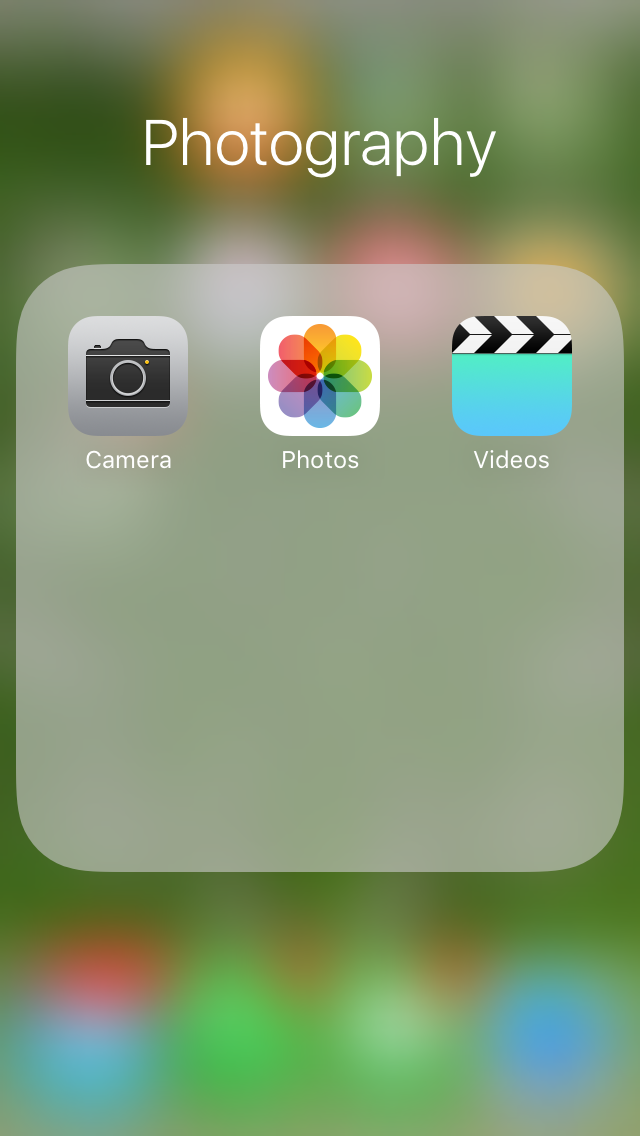This vertical image resembles a smartphone screen capture. The background is a soft-focus medley of colors—reds, greens, and oranges—suggestive of clustered Christmas lights on a green tree. The blurred lights contribute to a dreamy, festive atmosphere. 

Prominently displayed at the top center in crisp white lettering is the word "Photography." Below this title is a semi-transparent, pale white square with rounded corners, giving it an elegant, modern appearance. Inside this opaque box are three app icons arranged in a neat row from left to right.

The first app icon is labeled "Camera," featuring a minimalist black and white camera graphic with the lens facing forward. The second icon, "Photos," showcases a vibrant color wheel with large, oval petals that form an eight-sided diamond pattern in the center, accentuated by a small white circle. The third app icon, named "Videos," depicts a clapperboard used in filmmaking, characterized by its turquoise blue base and alternating black and white striped top.

This detailed image captures the essence of a functional and aesthetically pleasing smartphone interface, set against a backdrop of festive bokeh lights.